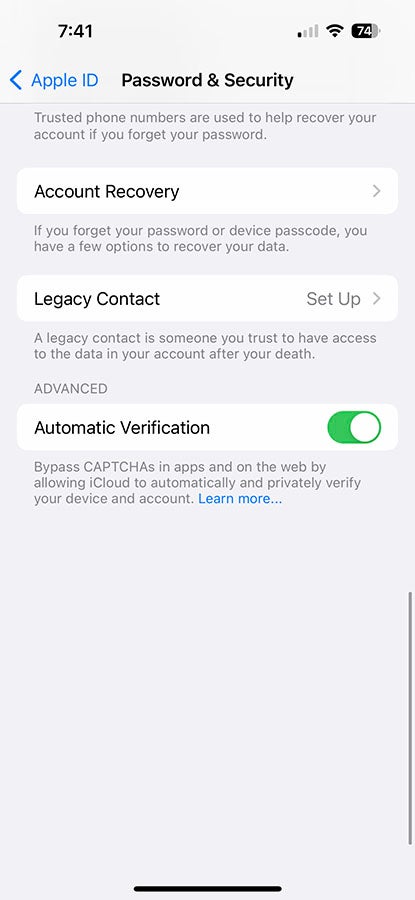**Image Description:**

The image appears to be a screenshot of an iPhone's settings related to Apple ID, Password, and Security. 

- At the top of the screen, the battery icon indicates a 74% charge.
- The Wi-Fi icon is visible, suggesting the device is connected to a network.
- The screen displays various configuration options, most notably related to trusted phone numbers used for account recovery. The text emphasizes the importance of these numbers in recovering the account if the user forgets either their password or device passcode.
- The section for "Apple ID Password and Security" is visible but grayed out, indicating that these settings are not accessible in the current view.
- Further down, there is a section labeled "Legacy Contact Setup." This feature allows the user to designate a trusted individual who can access the data on their device in the event of their death.
- There is also an "Automatic Verification" section with a green toggle switch. This setting enables the device to bypass captchas in apps and on the web by allowing iCloud to automatically and privately verify the user's device and account.
- Additional information can be accessed through a "Learn More..." link at the bottom of this section.
- The background of the screen appears to be dark or in dark mode, providing contrast to the white text and green toggle.

Overall, the screenshot captures various security and verification features designed to protect the user's Apple ID and simplify device access and data recovery.